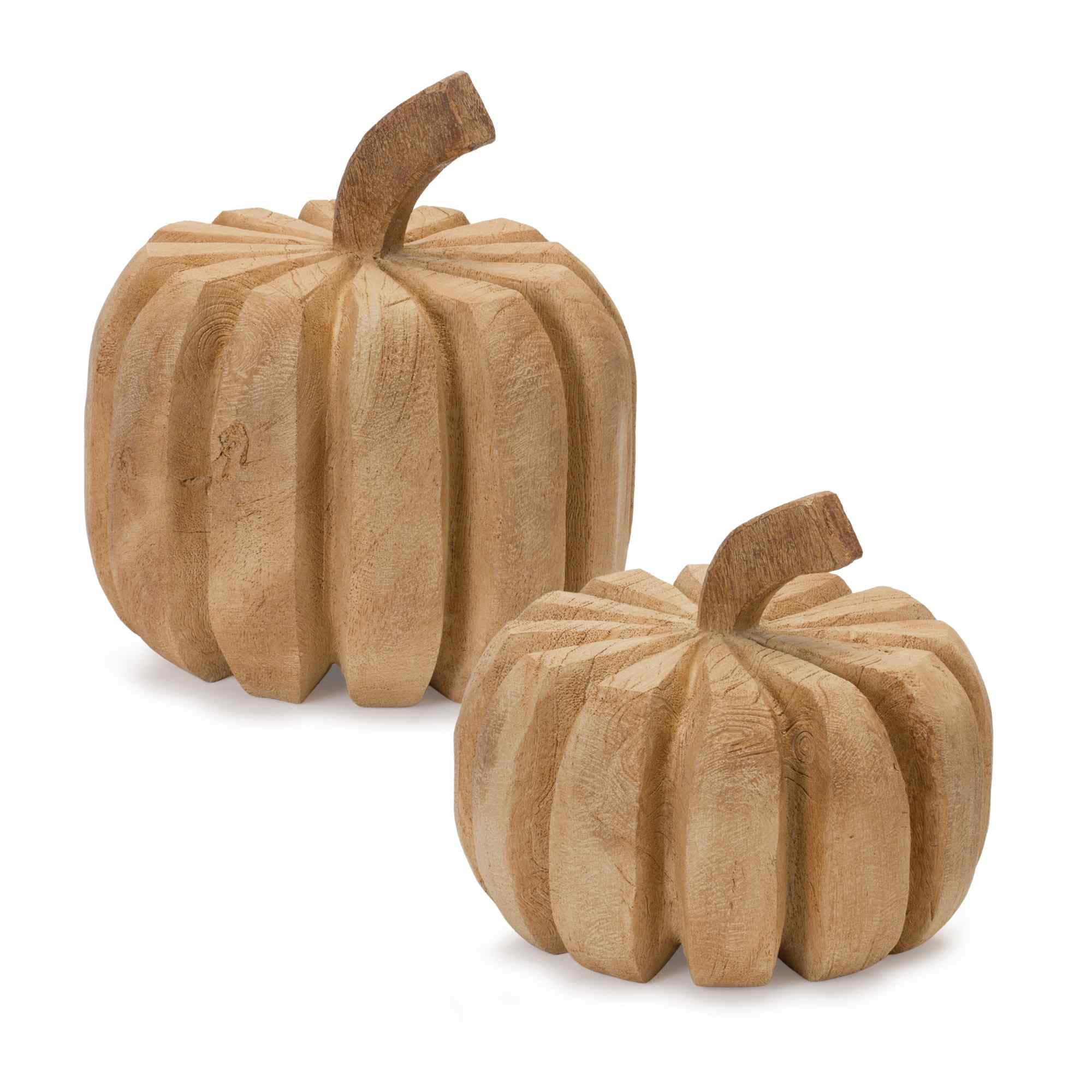This image showcases two wooden, intricately carved pumpkin-shaped sculptures. The larger pumpkin is positioned at the top left corner of the image, boasting a robust, rounded form. Both pumpkins feature elegantly curved stems that sweep downward to the right, enhancing their lifelike appearance. The front of each pumpkin seems to face the lower left corner of the image, creating a dynamic visual perspective. The smaller pumpkin, placed at the bottom right, mirrors the shape and design of the larger one but is more slender and compact. Together, these wooden pumpkins exude rustic charm, showcasing skilled craftsmanship and artistic attention to detail.